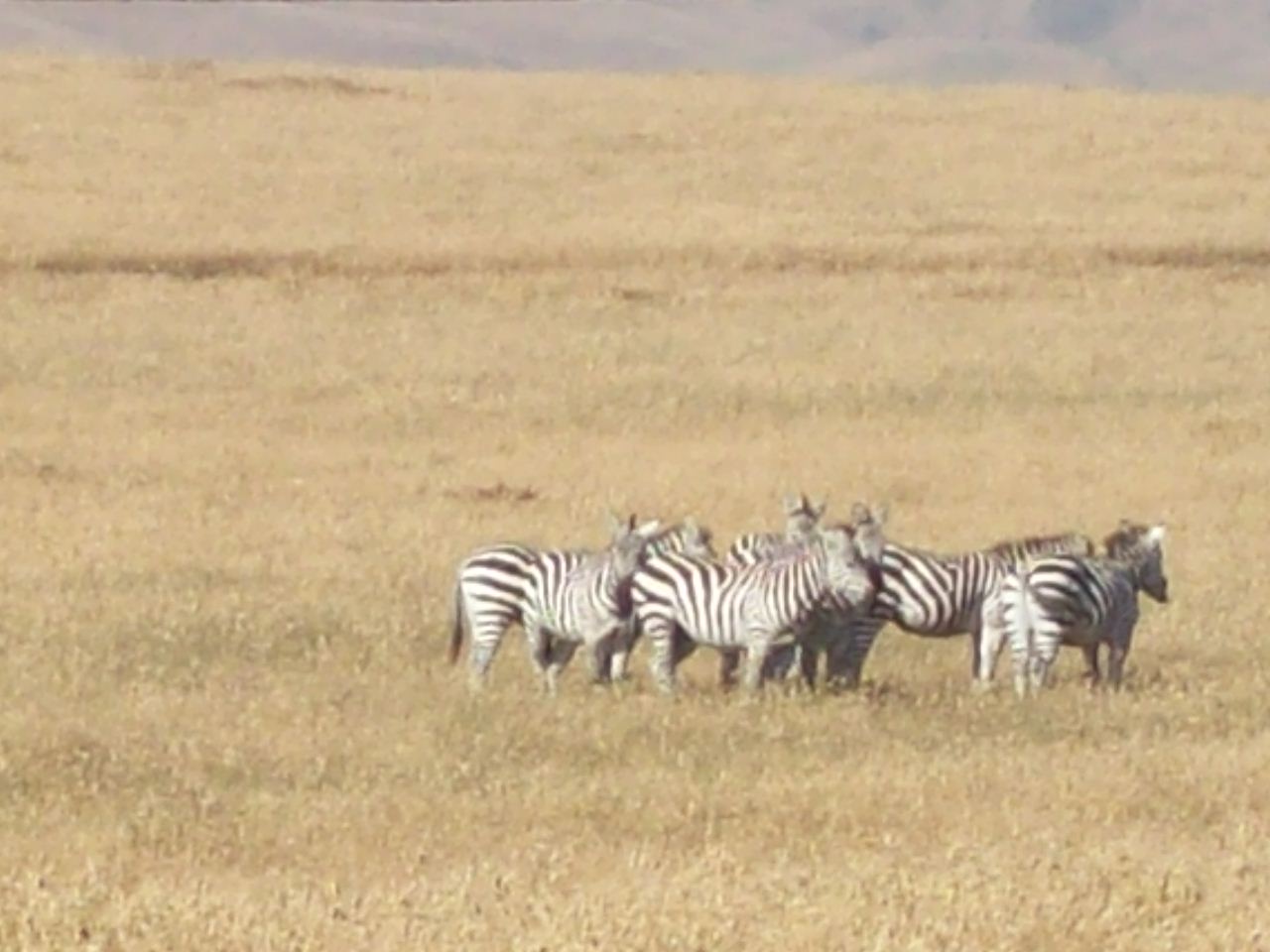This wildlife photograph, likely taken by an amateur on safari, captures a herd of zebras grazing in a sprawling savanna or grassland under bright, sunny skies. The image is in color but appears grainy, overexposed, and slightly out of focus. The terrain dominates the frame, featuring mostly yellowish-brown, dried grass with sporadic green streaks, suggesting a parched landscape. In the background, along the top edge of the photo, faint browny-grey foothills or mountains are barely visible.

The zebras occupy the bottom third of the composition, with about seven or eight animals grouped closely together, mostly facing towards the right side of the image. A couple of zebras in the back turn their heads towards the camera, while one at the rear rests its head on the rump of another. The herd's tight clustering could indicate either a defensive stance against a nearby predator or a natural behavior for mutual comfort and protection. Despite the technical flaws in the photo, the scene vividly conveys the essence of untamed wildlife in its natural habitat.